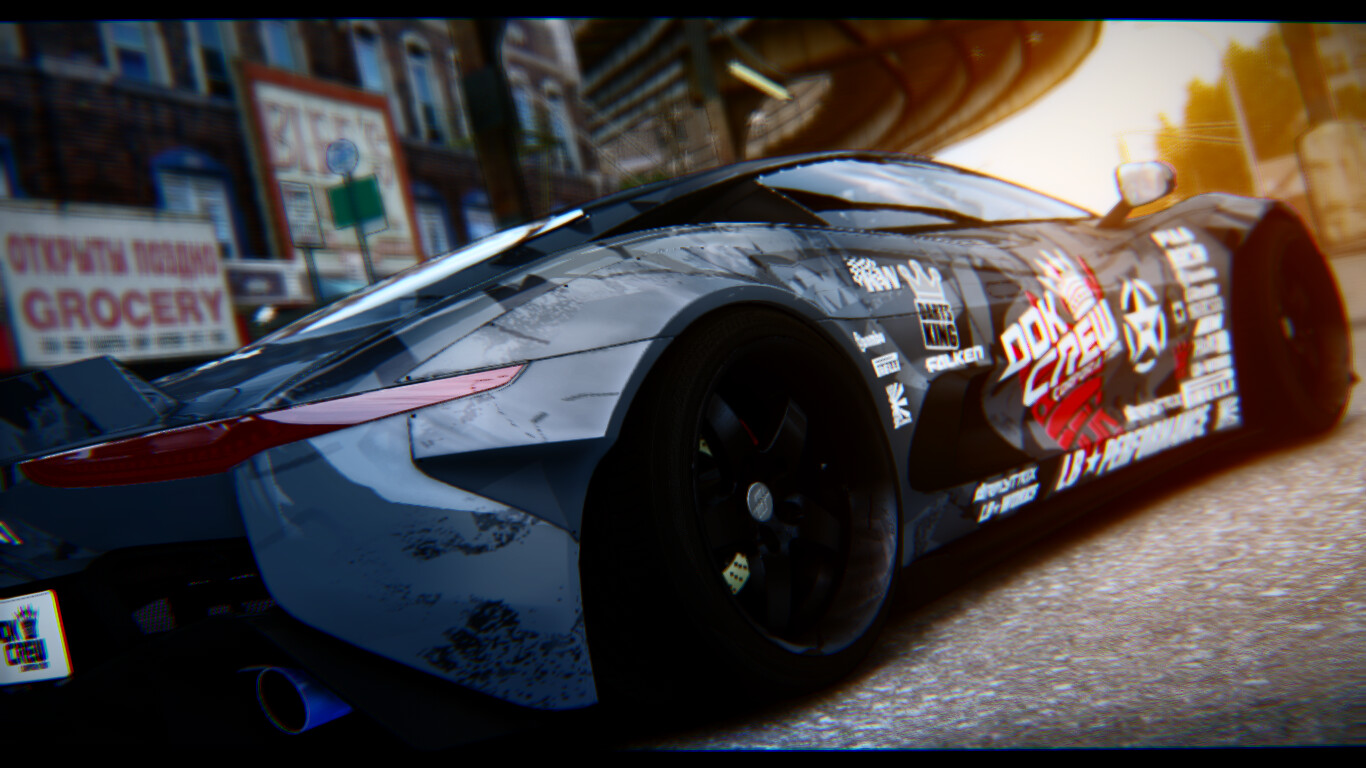This image showcases the side view of a futuristic-looking race car, reminiscent of an advanced European sports car. The vehicle is primarily black, featuring a large advertisement for something named "Dock Crew" on the passenger side door, with the text in bold white and outlined in red. Additional smaller logos in white, including one for "L.B. Performance," are scattered across the car's side. The backdrop includes a street scene with various local shops and a grocery store, along with glimpses of trees and a bright, sunny sky. A bridge, likely for a railway or subway, spans above the car, suggesting a bustling urban environment. The overall setting appears to be from a video game, given the hyper-realistic yet slightly stylized appearance.